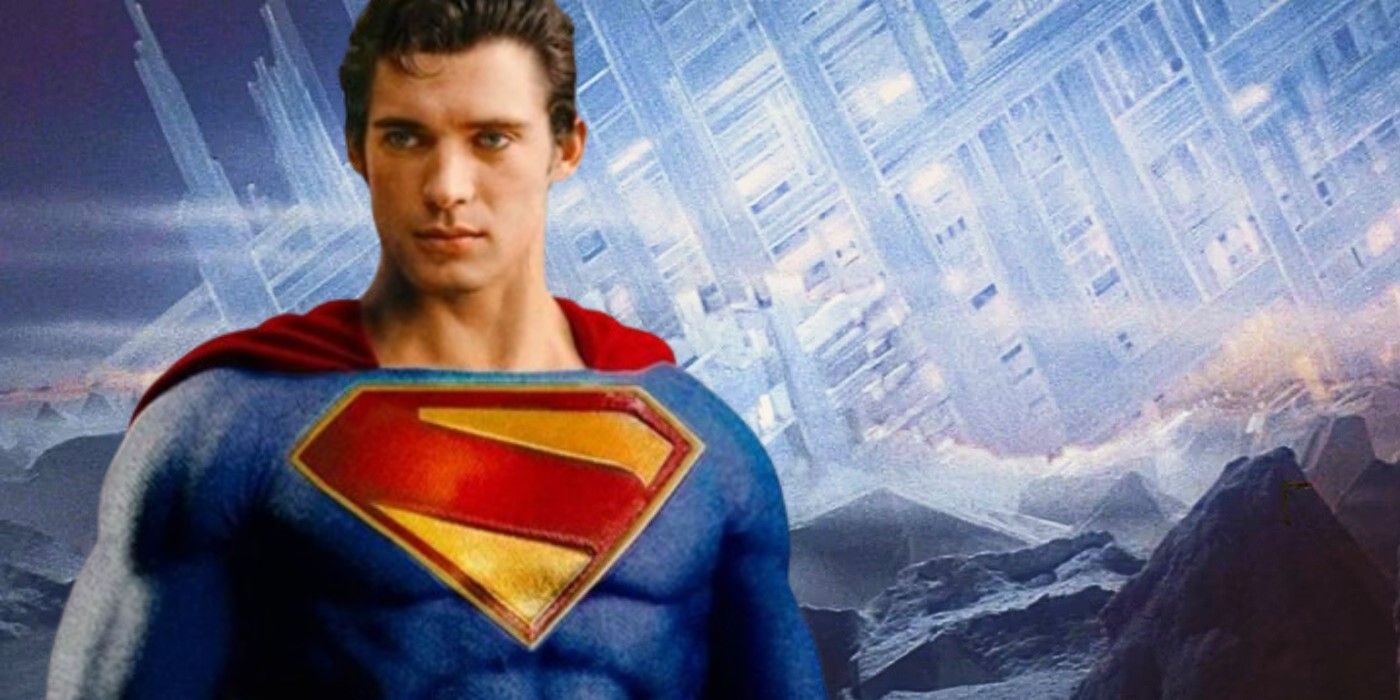In this photorealistic digital artwork of Superman, we see the iconic superhero standing on the left-hand side of the image, captured from the chest up. He boasts a muscular build, clearly visible through his form-fitting blue top, which prominently features the classic diamond-shaped, yellow emblem with a red "S", albeit with the top and bottom strokes of the "S" blending into the frame of the traditional pentagonal logo. Superman has short, slicked-back brown hair with a signature forelock curling onto his forehead, light-colored eyes, and slightly asymmetrical, low-set eyebrows—one thicker than the other. His red cape emerges from behind his neck and tucks seamlessly under his shirt. Superman gazes intently off to the left, his eyes slightly narrowed, as if focusing on something in the distance. The background presents an otherworldly, angular landscape, composed of what appears to be rocky outcrops or mountains. These formations are set against a surreal sky dominated by a grayish-white, almost icy lattice-like pattern, interspersed with streaks of light blue, suggesting a scene that defies earthbound realities.